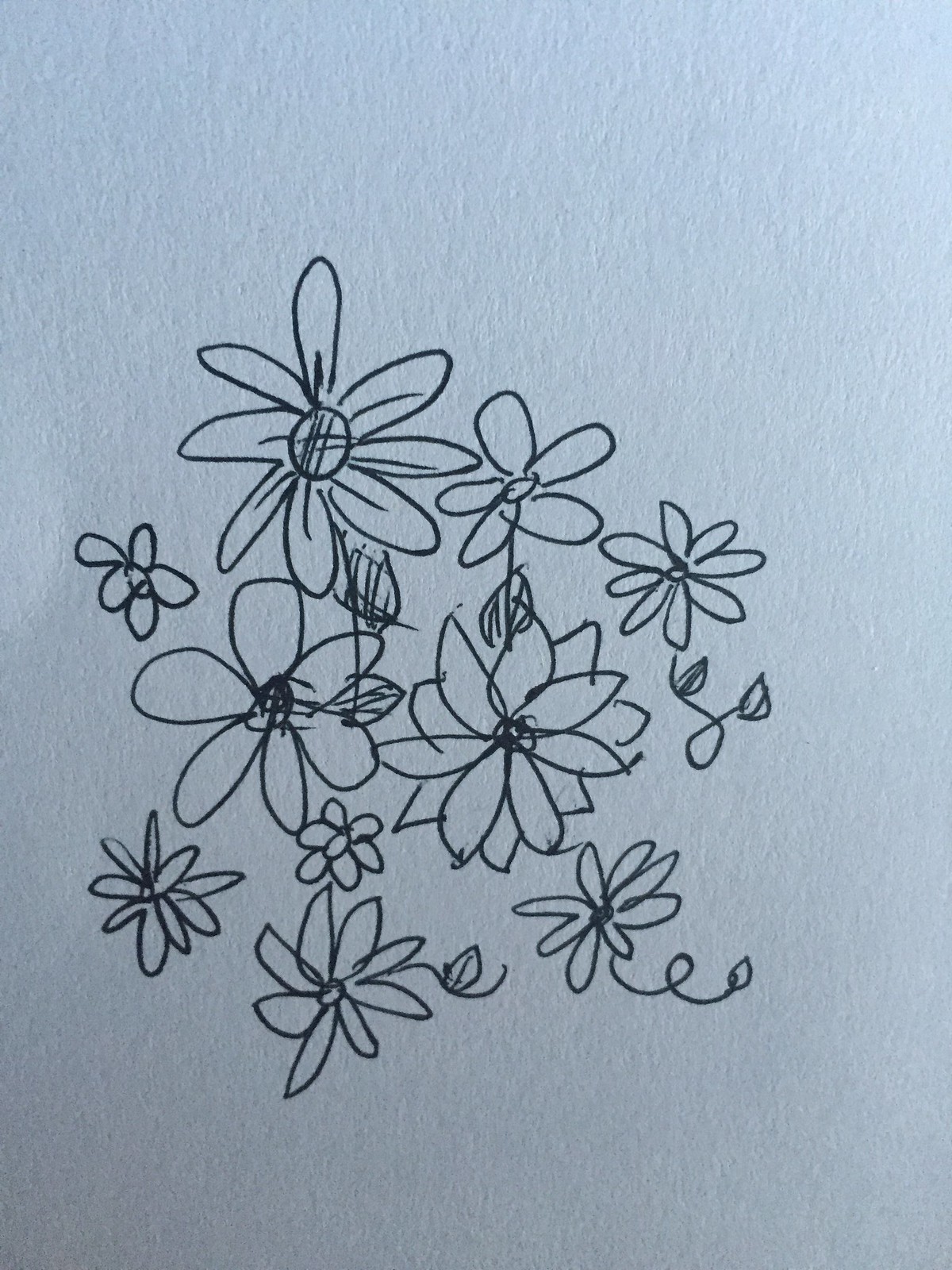A detailed black marker illustration of clustered daisies fills the entire frame of this plain piece of paper. The flowers, meticulously drawn, showcase a variety of petal arrangements; with some daisies featuring as few as five petals while others boast a dozen, some even arranged in a distinctive double row. The blossoms, ranging in size from small to considerably larger, are tightly grouped at the center of the page, creating a visually engaging focal point. This harmonious cluster is further accentuated by a few delicate, curling stems and leaves, adding a touch of organic flow to the composition.